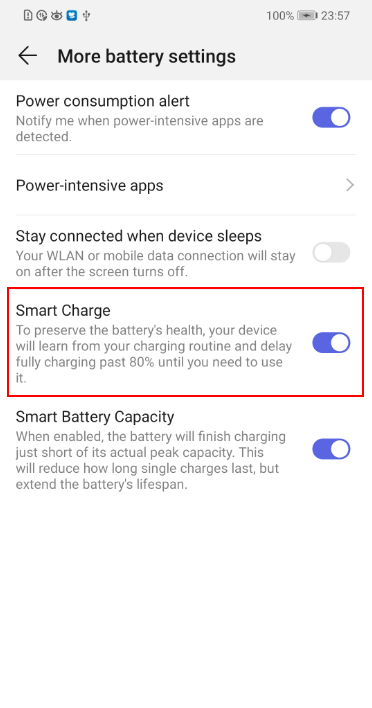The image showcases a screenshot taken on a cell phone, focusing on the "More Battery Settings" menu. At the top-left corner of the screen, a grayish background displays the title "More Battery Settings." Along the top edge of the screen, various icons are visible. On the right side, the battery icon shows a 100% charge, and the time is displayed as 23:57.

Below the title, the settings menu is organized with options listed on the left and corresponding sliders on the right, allowing users to toggle each setting. The first setting, "Power consumption alert," is enabled, indicated by a blue slider with a white knob positioned to the right. The "Power intensive apps" option follows, accompanied by a right-pointing arrow, suggesting further details can be accessed.

Further down, the "Stay connected when the device sleeps" option is currently turned off. The "Smart charge" feature is activated, highlighted by a red rectangular border surrounding the section and its explanation. At the bottom of the screen, the "Smart battery capacity" setting is also switched on.

This detailed and organized display illustrates the various battery management options available on the device, providing a clear and comprehensive view of the user's current power settings.